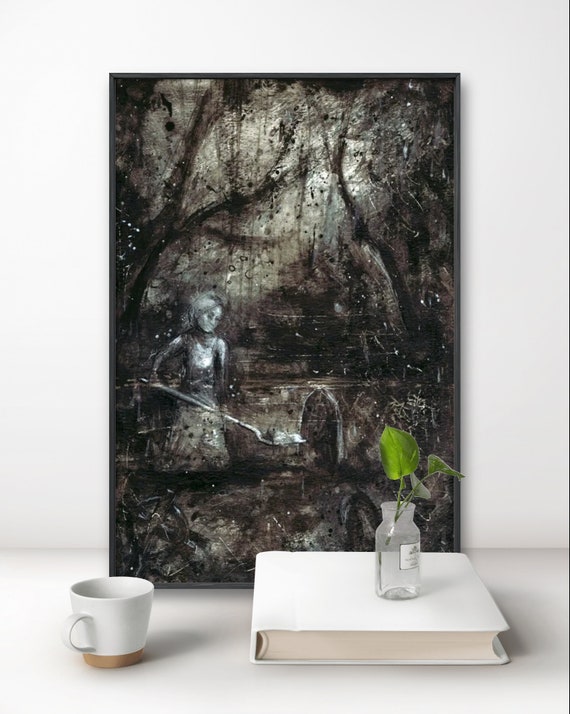The image captures a moody and dark painting leaning against a pristine white wall, set on an equally white tabletop. The artwork, framed in black, vividly depicts a dense, wooded forest with a murky, swamp-like atmosphere. Dominantly shaded in black and grey, the painting portrays a ghostly woman with long hair, dressed in simple clothing, caught in the act of shoveling dirt onto a grave in a graveyard scene filled with other tombstones.

In front of the painting, there is a simple white book with cream-colored pages, exuding a photo album feel. Resting on top of this book is a clear glass bottle, reminiscent of an apothecary jar, filled with water and housing a small sprouting plant with a few green leaves. To the left of the book, a white mug with a light brown base and a white handle holds coffee. The flat white surface and background of the wall enhance the striking contrast and dark moodiness of the artwork, creating an intriguing and atmospheric composition.